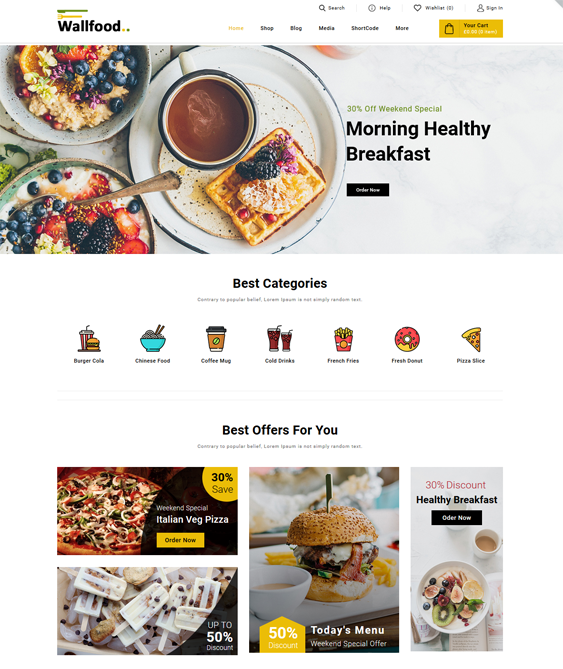The webpage features a prominent header with a green knife and fork icon, alongside the brand name "Wallfood" in black print, accompanied by a green dot, a yellow dot, and another green dot. To the right of the brand name, there is a search icon represented by a magnifying glass, followed by options for Help, a heart-shaped Wishlist icon, and a person silhouette icon labeled 'Sign In'.

Below the header, a navigation menu displays, with 'Home' highlighted in yellow print, and 'Shop', 'Blog', 'Media', 'Shortcode', and 'More' in black print. A yellow square icon containing a black shopping bag appears nearby, labeled 'Your Cart' in black text.

A banner beneath the navigation menu showcases plates of food with a green notification declaring "30% off weekend special." Below this, "Morning Healthy Breakfast" is written in black, and a black square labeled 'Order Now' in white print sits prominently.

The webpage continues with a section titled "Best Categories" on a white background. Though some smaller text under this header is blurred and illegible, discernible category icons include: Burger Cola, Chinese Food, Coffee Mug, Cold Drinks, French Fries, Fresh Donut, and Pizza Slice.

Further down, the section titled "Best Offers for You" presents various promotional images and graphics. Notable offers include an "Italian Wedge Pizza" with up to 50% discount, a "50% off Today's Menu" deal, and a "30% Discount Healthy Breakfast" promotion.